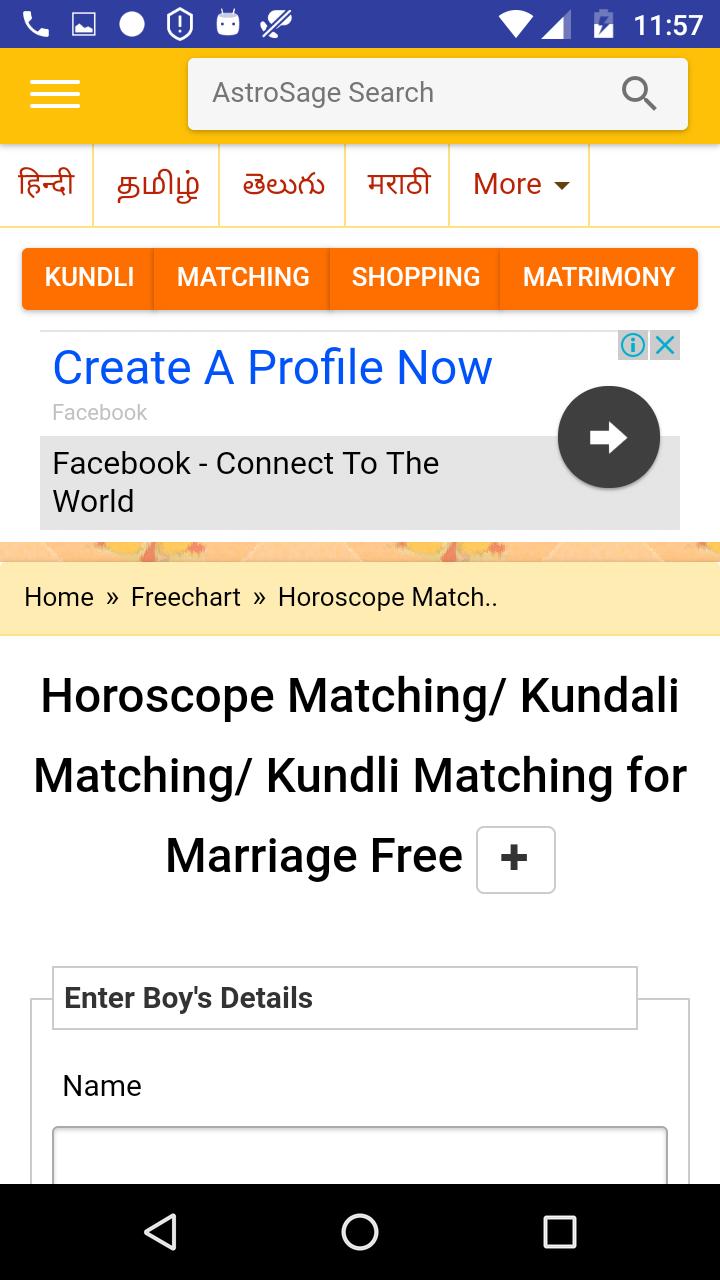This is a detailed screenshot taken on a phone, showcasing an application or website interface, likely named "Auto Astro Sage." At the top of the screenshot, a blue notification bar spans across, displaying various icons in white. On the left, a phone icon, a picture-like icon, a white circle, and three additional icons are visible. The right side of the bar notes the time as 11:57, alongside the battery percentage, Wi-Fi signal strength, and cell signal strength indicators.

Immediately below the blue bar, the interface prominently features an "Astro Sage" search bar, suggesting the potential app or website name. The content appears to be in Hindi, with five red links positioned below the search bar, the only readable link being "More," accompanied by a pull-down menu.

The interface proceeds with an orange navigation bar, divided into four sections labeled "Kundli," "Matching," "Shopping," and "Matrimony," all in white text. Following this bar, a Facebook advertisement appears.

Further down, another navigation bar is present, displaying "Home," "Free Chart," "Match," and "Scope." The subsequent section contains text advertising horoscope and Kundli matching services, specifically for marriage, described as free.